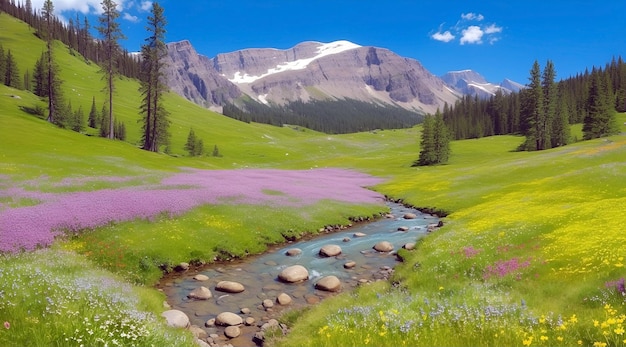The digitally generated landscape presents a vibrant alpine meadow with a stunning array of natural elements. Dominating the meadow are lush, bright green plains dotted with colorful flowers, prominently featuring lavender, blue, and yellow blossoms. A shallow, clear stream meanders through the center, its bed strewn with smooth, rounded stones and pebbles visible through the translucent water. Evergreen trees are scattered throughout the scene and densely cover the horizon, framing the view. In the background, towering, snow-capped mountains rise majestically against a deep blue sky adorned with wispy, scattered clouds, capturing a peaceful daytime ambiance.